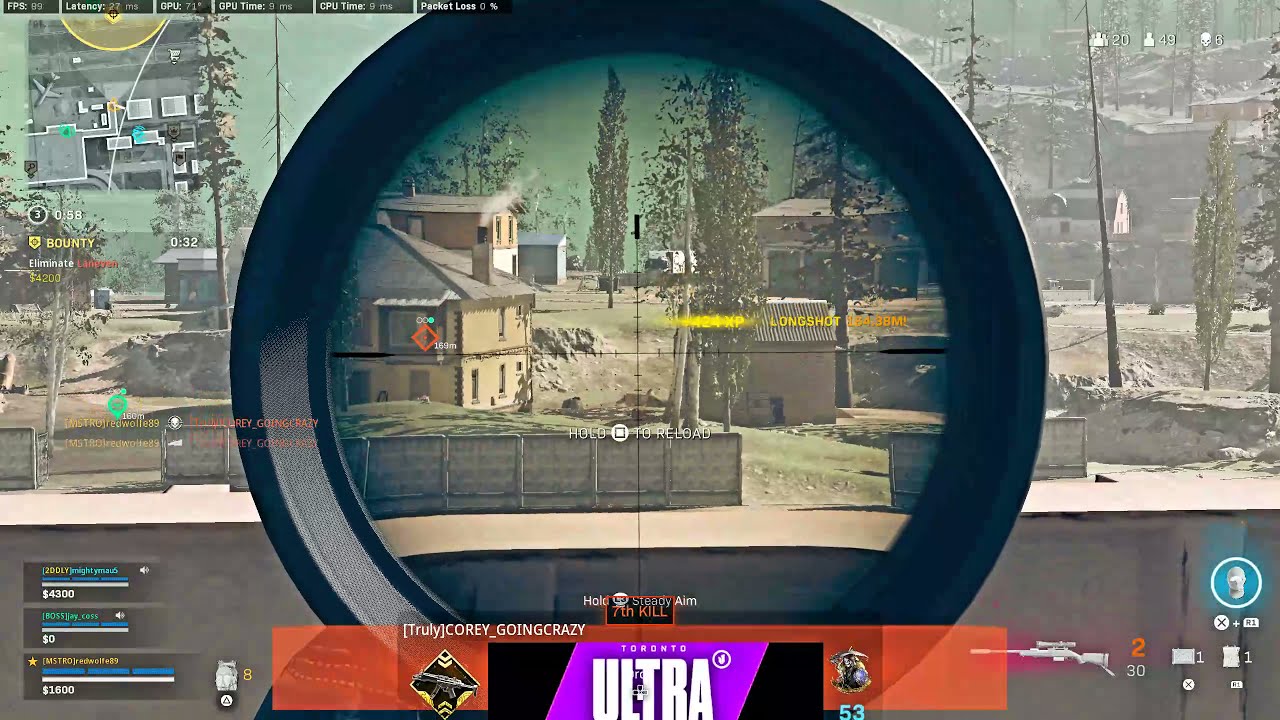This image captures a screen from a sniper video game in a first-person perspective. At its center is a black-bordered circle, which represents the sniper scope, displaying crosshairs that extend across the view, suggesting the readiness to take aim. The scene viewed through the scope reveals a village area with houses scattered around, bordered by pine trees, signages, and patches of sand on the ground. Snow is visible to the left side of the scene, adding to the environmental diversity. Other houses and tree-lined areas can be seen especially towards the right side.

Surrounding the main game view are various in-game tools and statistics: 

- The upper left corner is occupied by a mini-map.
- Bottom left displays health stats.
- Bottom right shows weapon selection options along with ammunition counts.
- The overall bottom section includes bars, numbers, icons, and progress indicators, with the words "Toronto Ultra" prominently displayed in a hot pink rectangle.

Additionally, the bottom section features the text "truly Corey_going_crazy" suggesting either a player name or a chat handle, and a red-lettered "7th kill" within a black rectangle, indicating the player's recent accomplishment in the game.